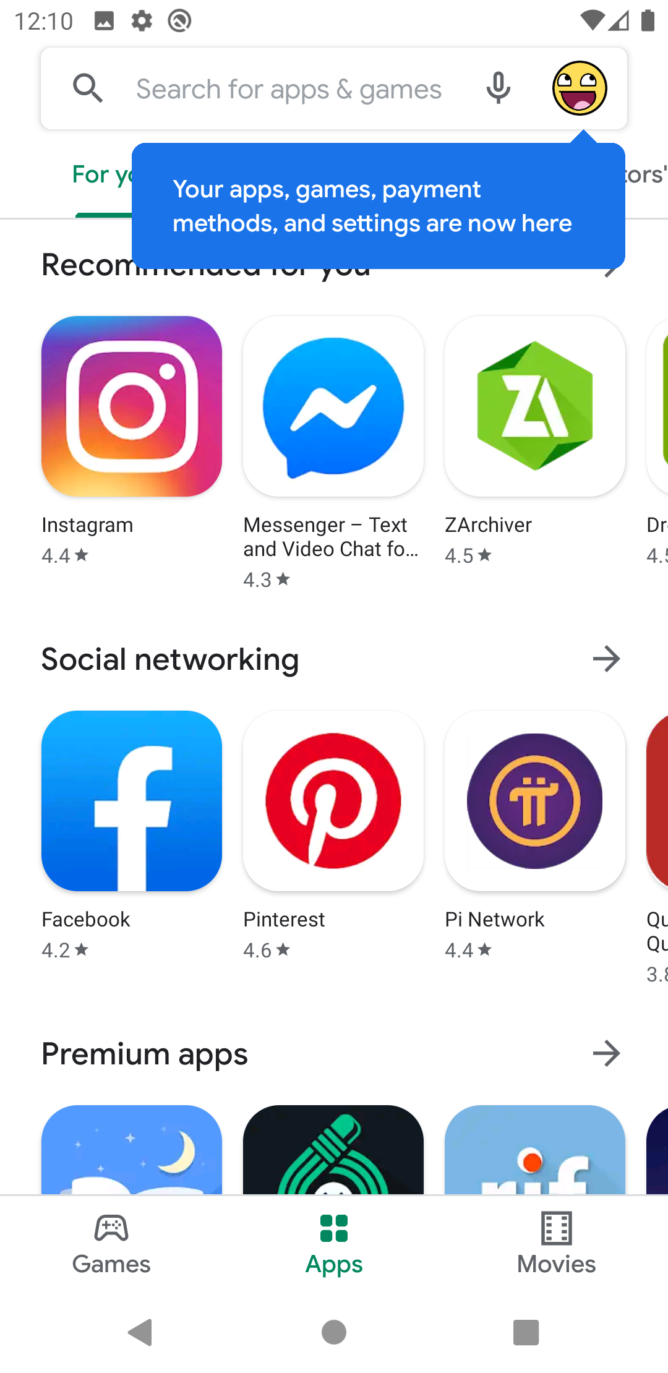This image is a detailed screenshot taken from the Google Play Store interface. At the very top, we see the phone's status bar displaying the current time as 12:10, followed by three small, gray icons: a photo icon, a settings icon, and an indistinguishable icon, all of similar size. To the right of these icons, we find a fully lit Wi-Fi indicator, a service bar indicator half full, and a fully charged battery icon.

Beneath the status bar lies the Google Play Store search bar, featuring a magnifying glass icon on the left, placeholder text reading "Search for apps & games," and a microphone icon on the right. Beside the microphone, there's a smiley face icon with a blue speech bubble stating, "Your apps, games, payment methods, and settings are now here." Partially obscured behind this bubble are additional text tabs, showing possibly more navigational options.

Continuing downward, we observe app recommendations by Google Play, organized into horizontal sections with prominent titles. The first section, titled "Recommended for You," presents apps such as Instagram, Messenger, and ZA Archiver, each accompanied by their ratings. Below, a section named "Social Networking" includes apps like Facebook, Pinterest, and Pi Network, along with their ratings. At the bottommost section titled "Premium Apps," the app icons can be seen, though their names aren't clear.

Toward the lower section of the screen, three navigation tabs are visible. The left tab labeled "Games," the middle tab labeled "Apps" (highlighted in green to show it's the current section), and the right tab labeled "Movies." Finally, at the very bottom, we see the device's navigation buttons: a triangle for the back button on the left, a circle representing the Home button in the center, and a square icon for accessing all apps on the right.